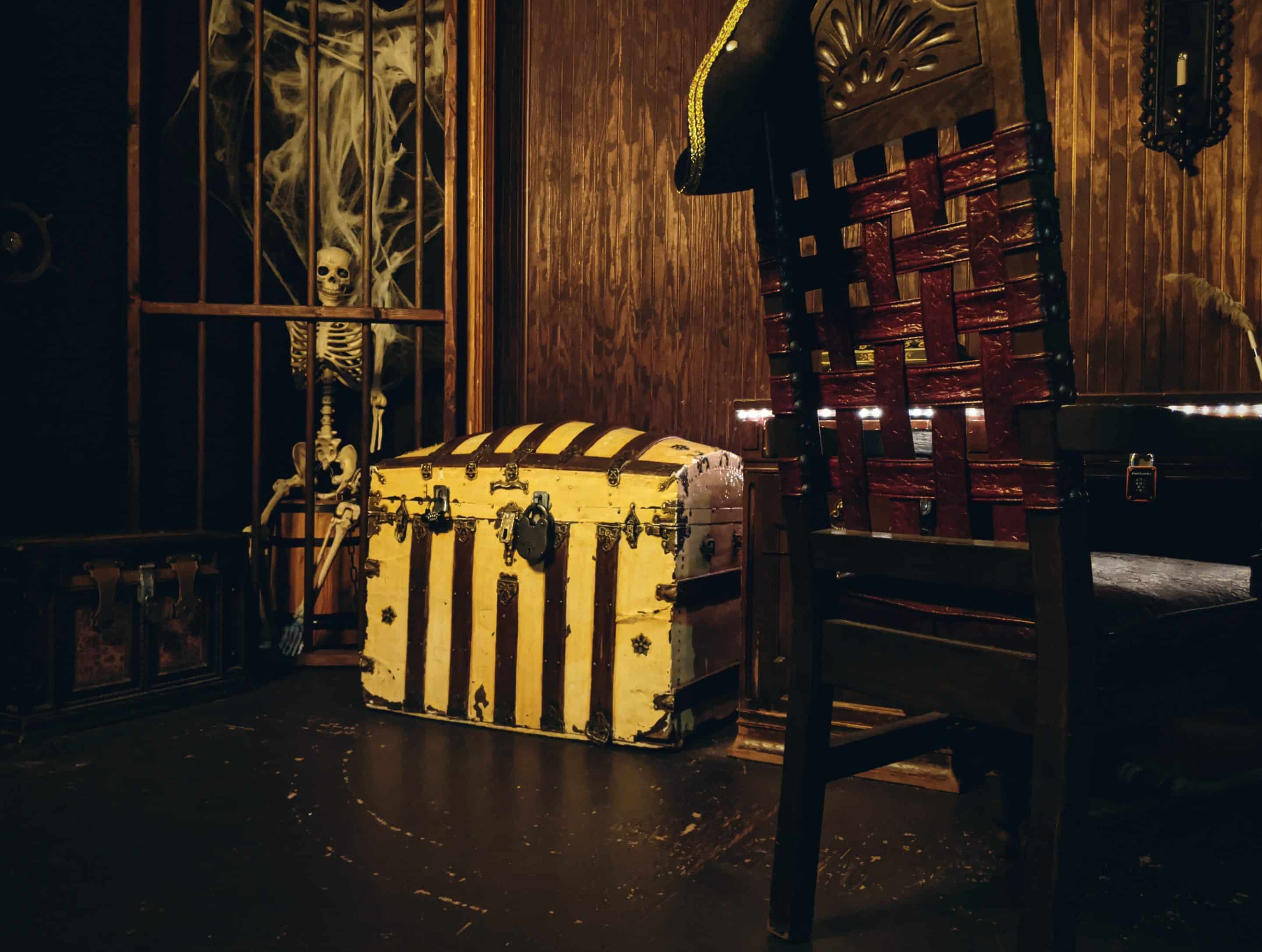The image captures a dimly lit, square room with a haunted house ambiance. Dominating the composition, a large, old chest sits at the center, characterized by its light brown wood, weathered appearance, and black/yellow striped pattern. The chest is secured with two padlocks, one smaller and one larger, emphasizing its antiquated, treasure-like essence. To the left, a gold-barred jail cell contains a white skeleton perched atop a brown barrel, draped in a weave of spiderwebs that add to the eerie, Halloween-like atmosphere. The room's right side features a dark wooden wall that extends to the middle top, accentuating the vintage feel with its mix of dark and medium brown panels. In the foreground, a dark wooden chair with a wicker backing stands by a wooden table; this vignette is completed with a black hat adorned with a yellow hem hanging on the chair. The floor's dark tones, mingled with gray curved scratches, contribute to the overall worn, historic ambiance.